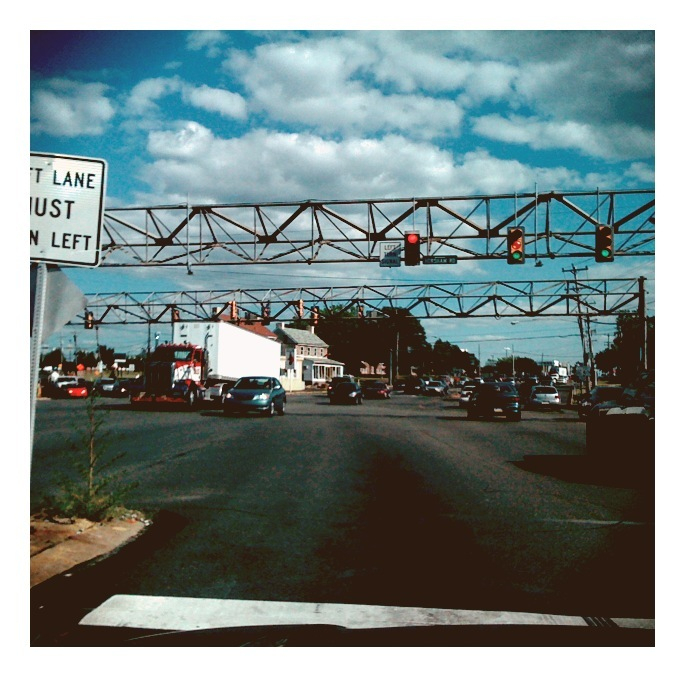This photograph captures a bustling traffic scene from the vantage point of a moving car. In the foreground, there is a traffic sign partially readable as "Left Lane Must Turn Left," and a series of horizontally mounted black rectangular traffic lights with circular indicators: one displaying red, and two showing green. The road is a worn blacktop with visible wear and tear, and a dividing line. Numerous cars, including a bluish-green one and a large red and white semi-truck with a white trailer, traverse the road. The scene is framed by a white house or building surrounded by lush green trees in the distance. The sky above is light blue, filled with dark gray wispy clouds and white patches. Additional traffic lights are visible on the far left. On the other side of the road, traffic appears to be heavy, showcasing a mix of passenger cars in various shades from silver to dark. Overall, the image captures the intricate details of a busy intersection under a partly cloudy sky.